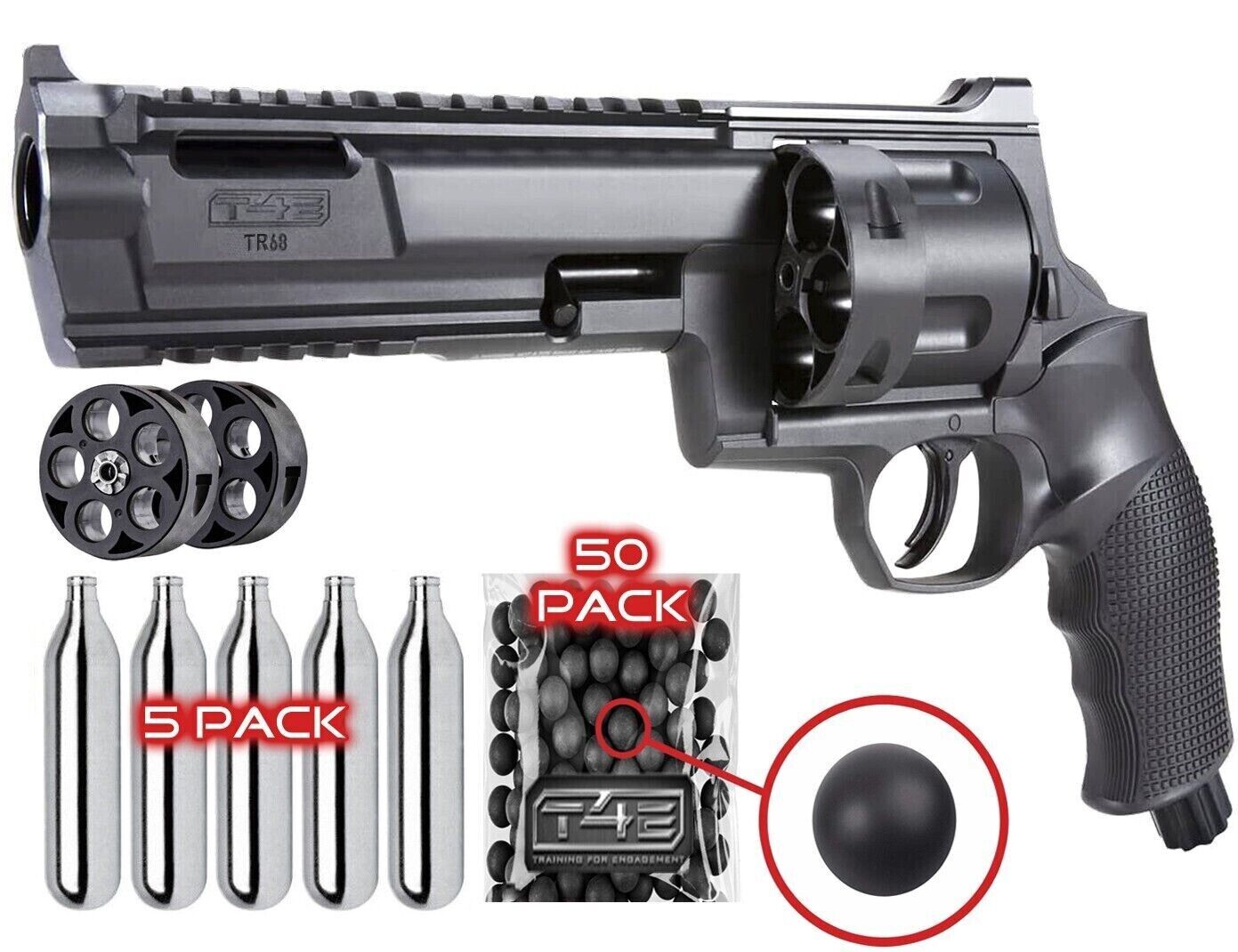This image features a detailed advertisement of a revolver-style airgun, oriented in a horizontal rectangle typical for online sales listings. The centerpiece of the image is a dark gray to matte black handgun marked with "T4E" at the tip of its barrel and "TR68" below that. The gun's magazine is slid out, revealing that it is empty. Beneath the gun are two additional cylindrical objects likely intended to hold air cartridges.

To the right of the airgun, there is a five-pack of silver, bottle-shaped air cartridges. Next to these cartridges is a package containing 50 spherical pellets, labeled "T4E, Training for Engagement." The label is set against a red background with white lettering. One of the pellets is highlighted in a blown-up inset, circled in red for emphasis. The pellets are depicted as black or dark gray, contributing to the overall professional aesthetic of the setup. The image, with its meticulous presentation, appears designed for promotional or retail purposes, showcasing the gun and related accessories in a clear and informative layout.